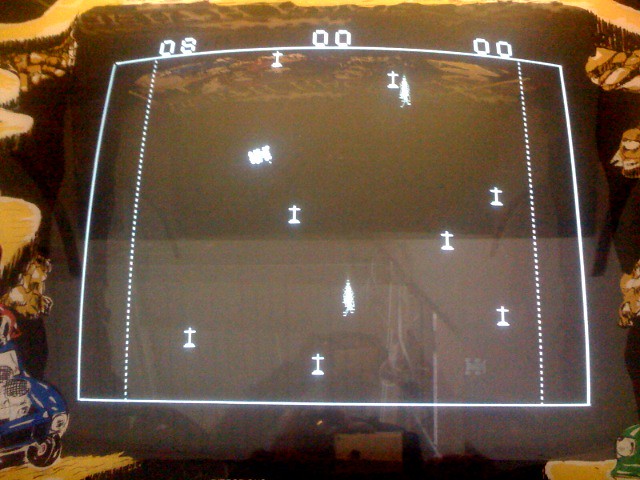A still image from a retro-styled video game is presented in this detailed description. The scene features stone textures framing the image on the left, right, and top sides. In the bottom left corner, the front end of a blue muscle car is prominently displayed with its hood open, revealing various white engine components. The left headlight, round and white, is clearly visible, along with the round, black left front tire seen from the inside.

In the center of the screen, which is outlined by a white rectangular frame, black background dominates, providing contrast for the game’s interface. White text is displayed at the top, showing "08" on the left, "00" in the center, and "00" on the right. The game screen is further populated with small bombs descending from the top, juxtaposed against rockets launching from the bottom in an attempt to intercept the bombs. The visual style is reminiscent of a 1980s Atari game, characterized by its pixelated graphics and simple, nostalgic gameplay elements.